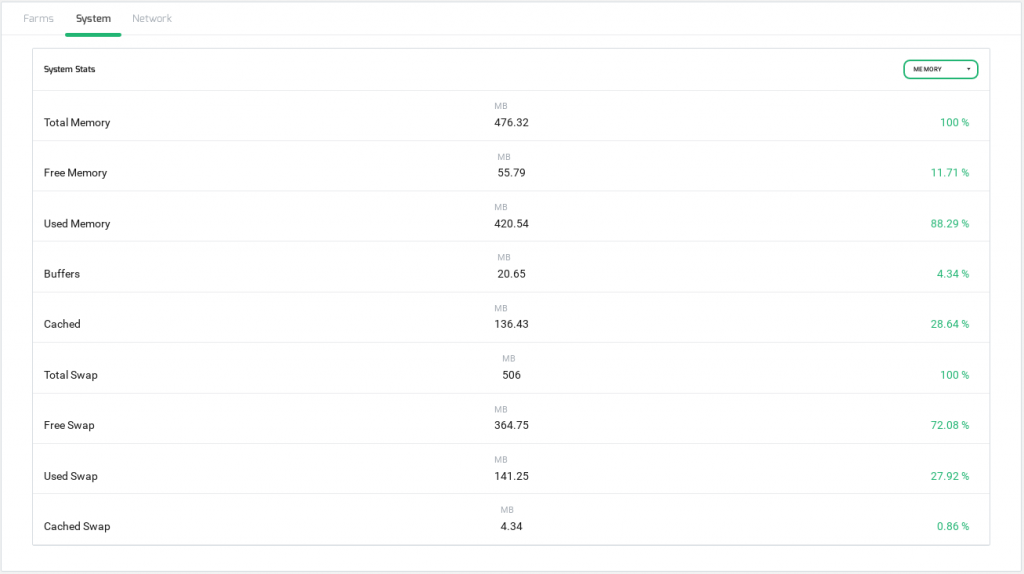This screenshot captures a detailed view of a computer system monitoring software interface. The background is completely white, creating a stark contrast with the black fonts used throughout the display. The top of the interface features three clickable sections: "Farms," "Systems," and "Network." In this image, the "Systems" section is selected, indicated by an underlining green line.

On the left-hand side, a vertical column lists various system statistics. This includes:
- Total Memory
- Free Memory
- Used Memory
- Buffers
- Cached
- Total Swap
- Free Swap
- Used Swap
- Cached Swap

Adjacent to these labels, towards the middle of the interface, the memory usage values are displayed in megabytes. Further to the right, the corresponding memory percentages are shown, with all values highlighted in green to denote perhaps normal operating conditions.

In the upper area of the interface, there is a drop-down menu labeled "Memory," offering presumably more refined or additional options related to the memory statistics being displayed.

Overall, the interface provides a comprehensive overview of the system's memory status, combining clear, concise data presentation with an intuitive, well-organized layout.